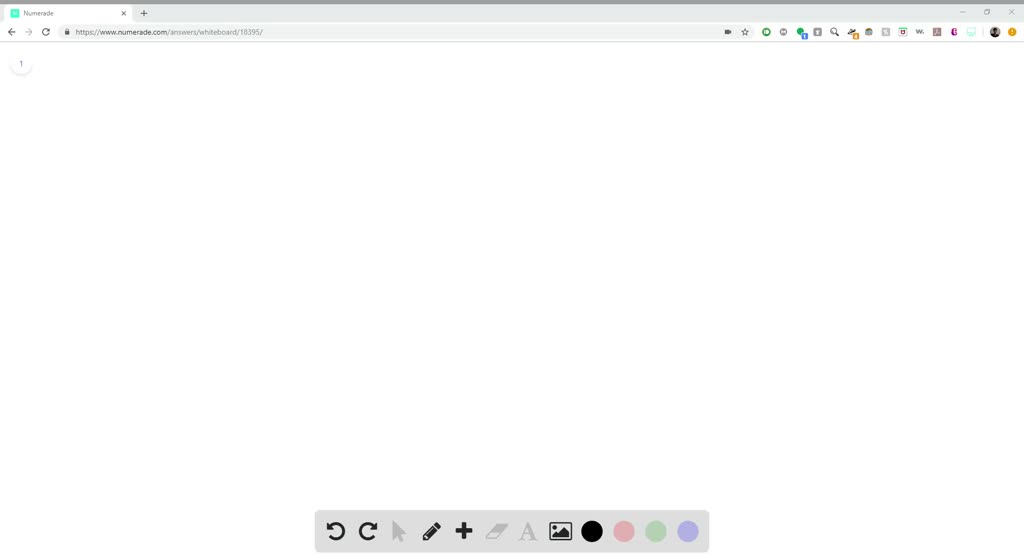Screenshot of the Numerade website interface:

The top section features a large green box with the Numerade logo, represented by a stylized letter "N." Below the logo, there are navigation buttons including a left arrow, a right arrow, and a reset button, all labeled clearly. Under these buttons, the web address "Numerade.com" is prominently displayed, along with the numeral "1," indicating the first step or page in a sequence.

As your eyes move down towards the bottom of the screen, additional functional buttons appear. These include dual arrows for refresh, a single arrow pointing upwards, an icon resembling a crayon accompanied by a plus sign, a phone icon, and a large capital letter "A." There is also an image icon displayed.

A palette of colors—black, pink, green, and lavender—is available, suggesting that users have the option to color or draw directly on the screen. This diverse array of tools and features implies a highly interactive and visually engaging user experience on the Numerade platform.